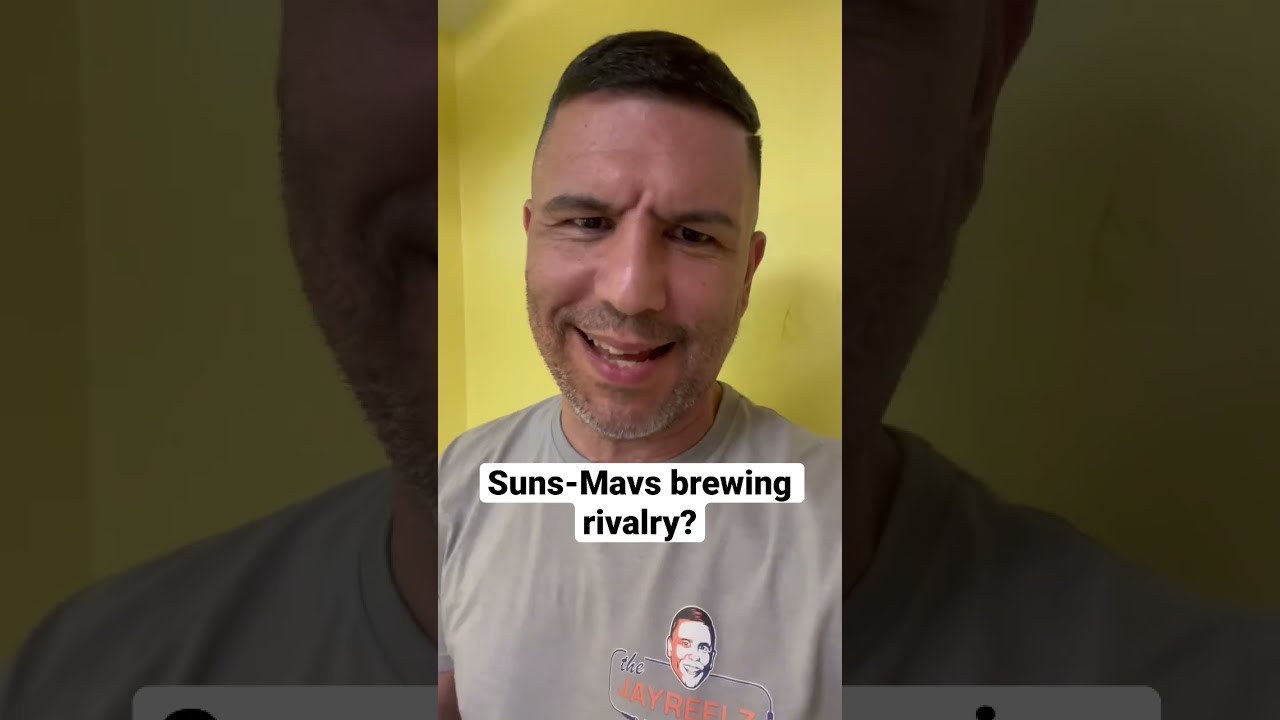In this portrait-oriented frame, likely from a TikTok or YouTube video, a white man dominates most of the image. He appears to be in his 40s, with dome-shaped brown hair and a neatly trimmed grey beard. He's wearing a grey t-shirt with a logo on the left side of his chest that reads "Jayreels," spelled J-A-Y-R-E-E-L-Z in black and white. The t-shirt also features an image of a human face as part of the logo. The man is mid-sentence, his mouth partially open, and he has an expression of incredulity. His right eye is slightly more open than the other. The solid yellow background adds a vivid contrast to the scene, which also has superimposed black text on a white background reading, "Sons-MAVS Brewing Rivalry?"